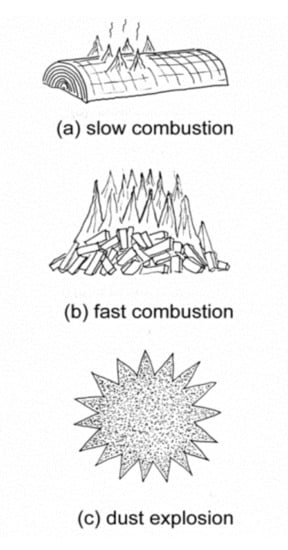This rectangular, black and white diagram, set against a light speckled grayish-blue background, illustrates three different types of combustion: slow, fast, and explosive. At the top (Option A), a half log with small triangles rising from its flat surface and three wavy lines above it is labeled "a" with the description "slow combustion," indicating a slower burn due to the log's size. In the middle (Option B), labeled "b" and described as "fast combustion," several small wood chips are shown stacked together with tall, thin flames emerging from them, representing rapid combustion. At the bottom (Option C), labeled "c" and described as "dust explosion," a sunburst symbol suggests an intense, explosive event.